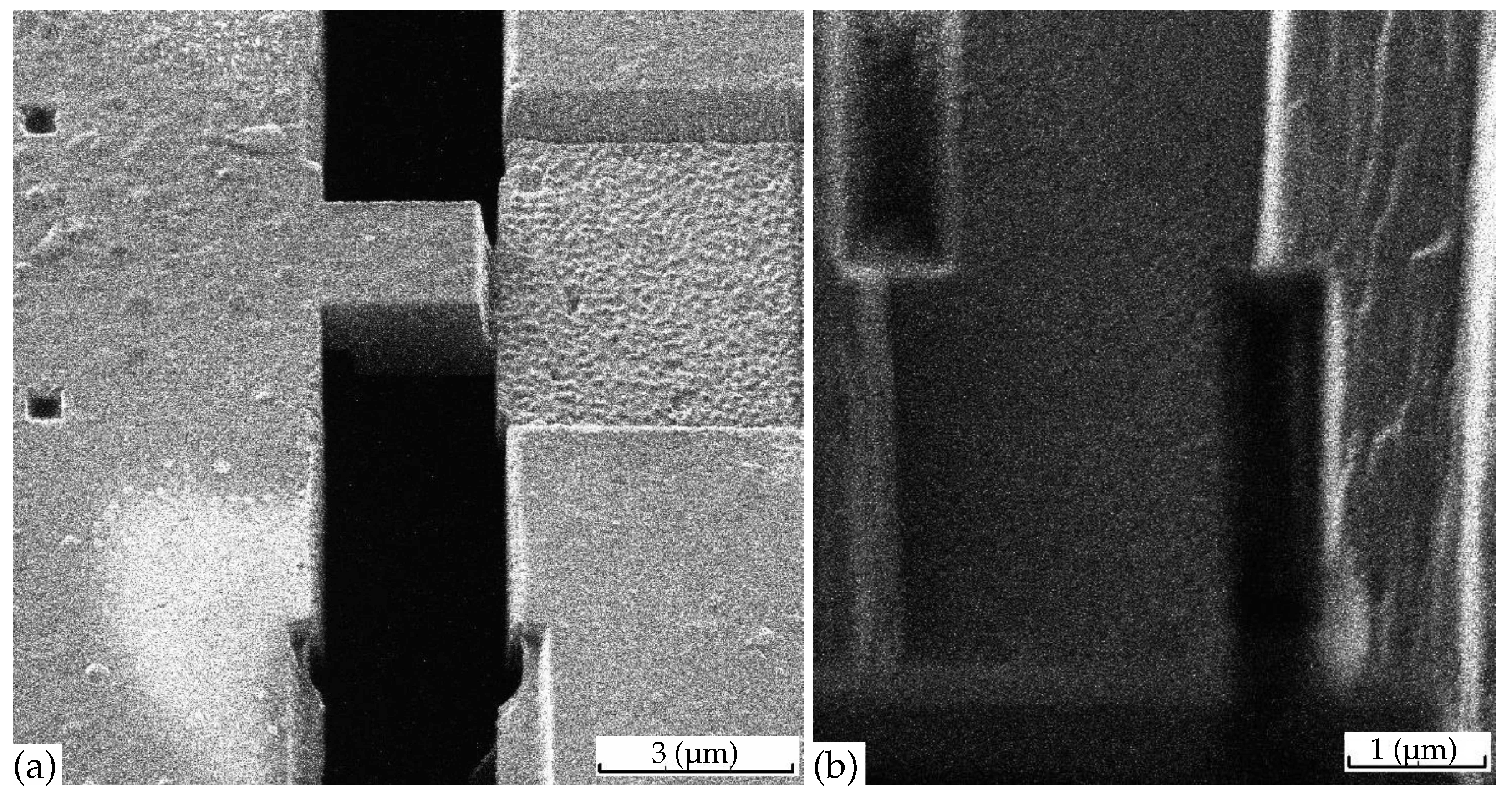This closely cropped image features two side-by-side grayscale photographs of textured materials labeled A and B, respectively. The left image (A) depicts a light gray, stone-like texture with a unique pattern that includes rectangular areas and suggests two connected pieces with a Tetris-shaped connector in the middle. This side also has black space around the structure, and at the bottom, it is labeled "A" in a white box, followed by "3 (UM)" with a measurement stick beneath it, also in a white box. The right image (B) portrays a contrasting dark gray texture with crinkled lines and a wood-like appearance. In the bottom left corner of this image, it features "B" in a white box, with "1 (UM)" and a measurement stick in another white box on the right. The overall grainy quality of the images evokes the appearance of industrial materials or machinery components, possibly captured under high magnification or specialized imaging techniques.